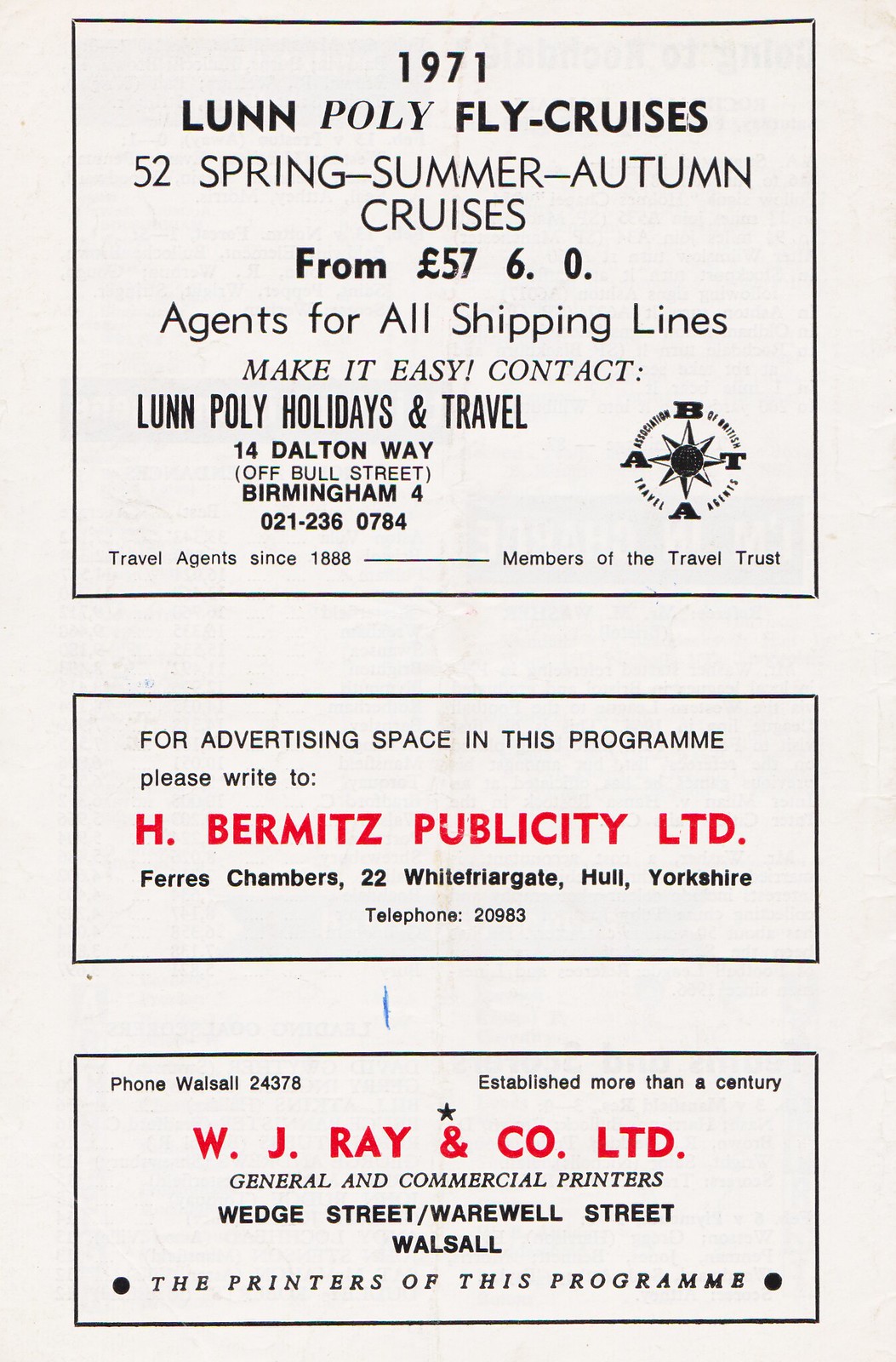This black-and-white scan, with selective red text, appears to be an insert from a magazine or flyer featuring three distinct advertisements. The top section promotes the 1971 Lunn Poly Fly Cruises, offering 52 spring, summer, and autumn cruises starting from £57.60. The advertisement emphasizes the agency's ease of access and contact details, indicating Lunn Poly Holidays and Travel located at 14 Dalton Way, Bull Street, Birmingham, with the phone number 021-236-0784 and notates they have been travel agents since 1888 and are members of the travel trusts. A compass logo with 'A', 'B', 'T', and 'A' at the cardinal points is prominently displayed. The second section invites readers to inquire about advertising space by contacting H. Bertsman Publicity Ltd. at Ferris Chambers, Wiregate Hall, Yorkshire, with the telephone 20983. The company’s name and address are highlighted in red. The third and final section advertises W.J. Ray and Co. Ltd., general and commercial printers located at Wedge Street/Warewell Street, Walsall. Their name is also printed in red and they are noted as the printers of the program.